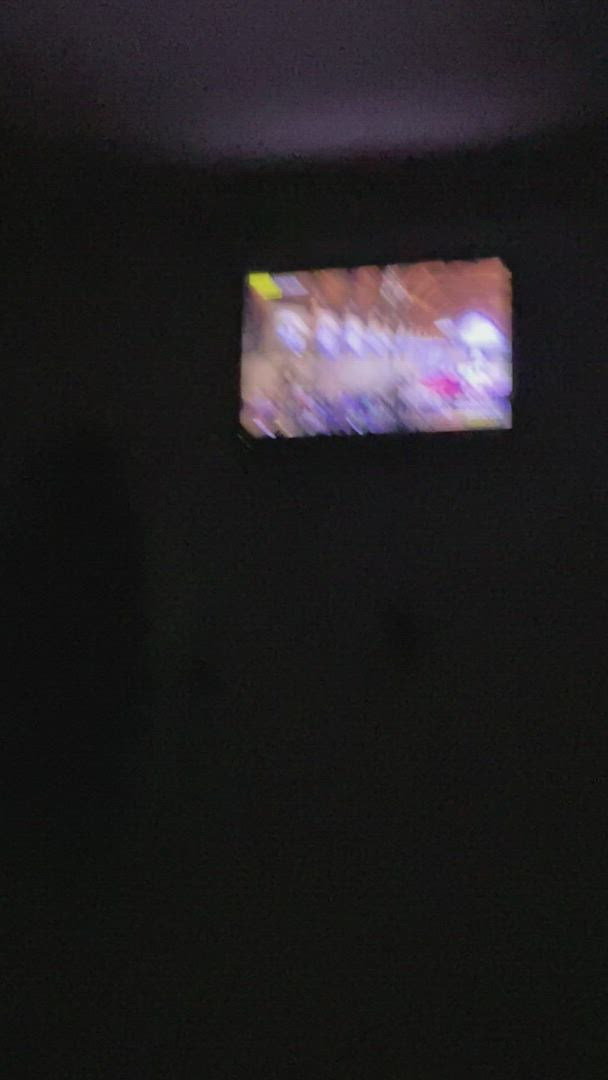The photograph is a very dark and highly blurry image of what appears to be the inside of someone's living room at night, with a TV screen glowing prominently. The TV, about 42 inches in size, is mounted on a wall slightly to the right side of the frame. The content on the TV screen is indistinguishable due to the blurriness, though it seemingly depicts an indoor scene that could be either the interior of a large church or a barn. The image itself has a brownish hue on top, transitioning to whites in the middle and occasional red patches towards the bottom, possibly indicative of people or objects. The room surrounding the TV is pitch black, save for some faint reflections of light on the white ceiling and walls, which are also blurred. The dark areas of the photo appear staticky and pixelated, suggesting that the camera was shaken during the capture. The screen itself has a small red blob in the center on the right side and a yellow blob in the upper left corner.